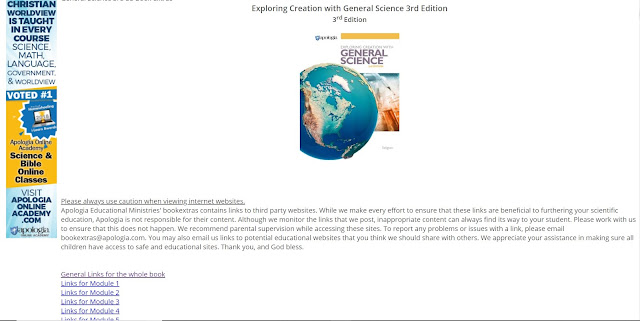The image features a vertical banner on the left-hand side with the following text elements: 

1. "Christian Worldview is Taught in Every Course" (bold font),
2. "Science, Math, Language" (lighter font),
3. "Government and Worldview."

Below this, a blue box highlights, "Awarded Number One Science and Bible Online Classes," and another blue box below it reads, "Visit ApologiaOnlineAcademy.com."

To the right of this banner, there is the main window content. Center-justified text states, "Exploring Creation with General Science Third Edition," with "Third Edition" mentioned again below. A visual showcases a book cover with an image of the Earth and the text "General Science." At the bottom, a difficult-to-read section advises, "Please use caution when visiting Internet websites."